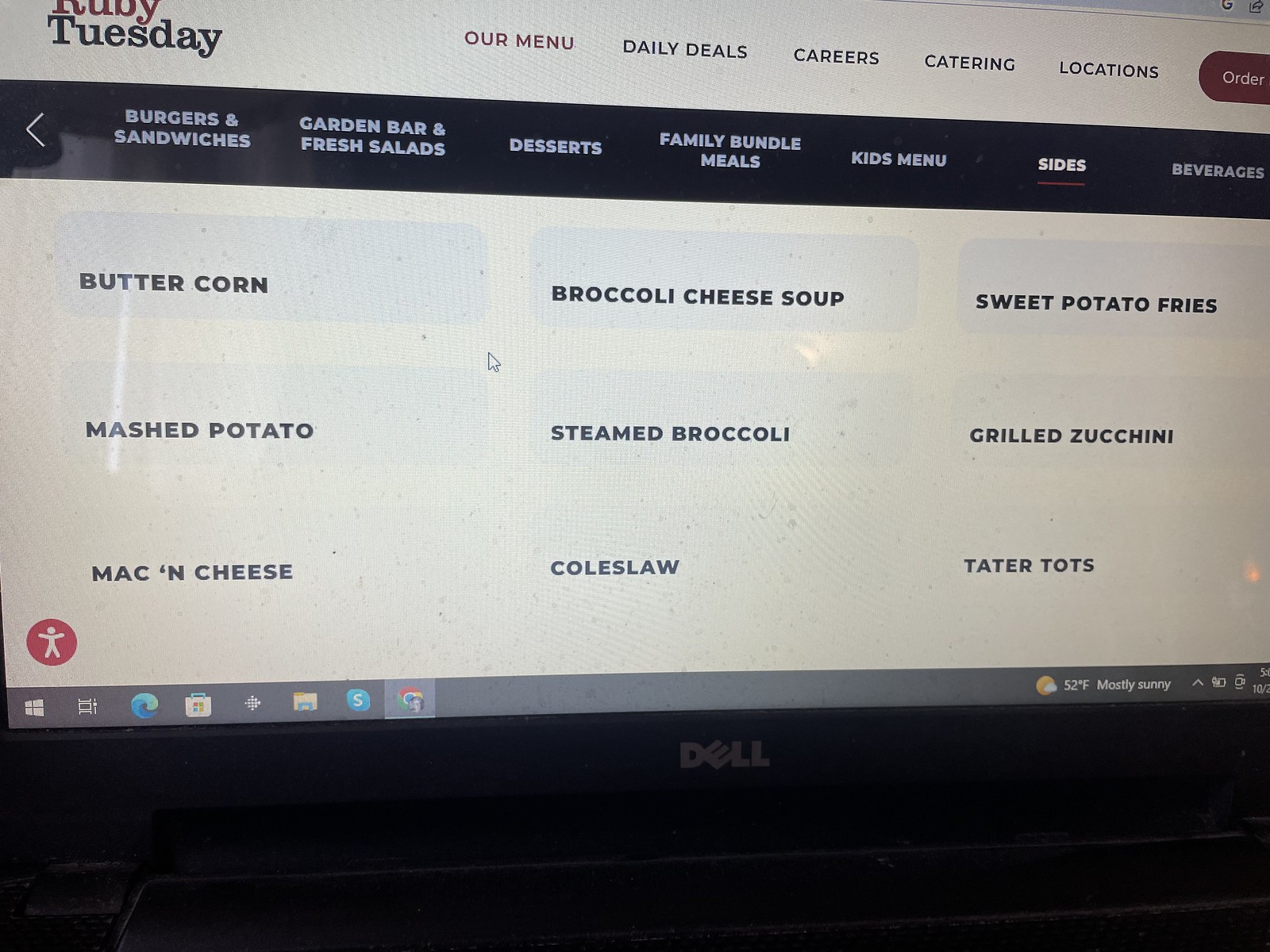The image showcases a computer monitor with a distinctly black-framed screen branded with a Dell logo at the bottom. On the top left of the screen, the Ruby Tuesday logo is prominently displayed, alongside a navigation menu featuring options like "Our Menu," "Daily Deals," "Careers," "Catering," and "Locations." To the right, a noticeable red oval button labeled "Order" is visible. 

Below this, a horizontal black stripe with white text categorizes different menu sections: "Burgers and Sandwiches," "Garden Bar and Fresh Salad," "Desserts," "Family Bundle Meals," "Kids Menu," "Sides," and "Beverages." The "Sides" section is highlighted, denoting its current selection with brighter white text.

In the lower portion of the screen, a large white space displays several gray rectangles, each containing bold black text listing side dish options: "Butter," "Corn," "Broccoli," "Cheese," "Soups," "Sweet Potato Fries," "Mashed Potato," "Steamed Broccoli," "Grilled Zucchini," "Mac and Cheese," "Coleslaw," and "Tater Tots." A mouse cursor is positioned slightly to the right and above the "Mashed Potato" option. Additionally, a small red circle with a stylized human figure, arms, and legs splayed out, is located in the lower left corner of the screen.